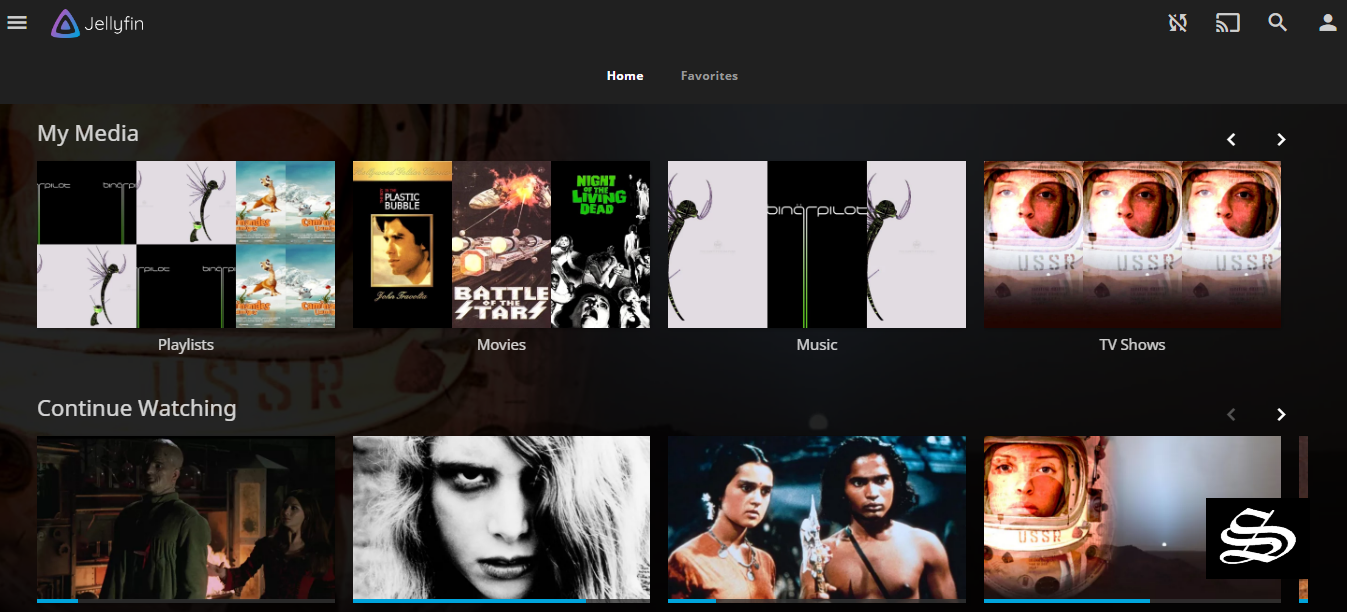A screenshot of the Jellyfin media server interface is displayed. In the upper left corner, three horizontal white lines denote the menu. Beside it is a triangle with another triangle inside, in a purplish-blue hue, followed by the word "Jellyfin" in white text. On the upper right, several icons are visible: two arrows split by a line, a square symbol with a Wi-Fi indicator at the bottom left, a magnifying glass for search, and a person silhouette representing the user profile.

Below the icons, navigation tabs read "Home" and "Favorites," followed by a section labeled "My Media." This section contains visual thumbnails of the user's media content, organized into categories. The "Playlists" category includes six images: two featuring a black figure on a white background, two that are predominantly black with a green line, and two with a bluish background and orange text.

In the "Movies" section, multiple movie thumbnails are displayed, though the text is mostly illegible due to size. Titles such as "Battle of the Stars" and "Night of the Living Dead" can be discerned.

The "TV Shows" section features a thumbnail of an astronaut with "U.S.S.R" written on it.

Finally, a "Continue Watching" section appears at the bottom. The first thumbnail shows a man and woman in a dark room; the second is a close-up, black-and-white image of a woman's face; the third shows a man and woman standing and looking at something; the final thumbnail repeats the image of the astronaut from the TV Shows section.